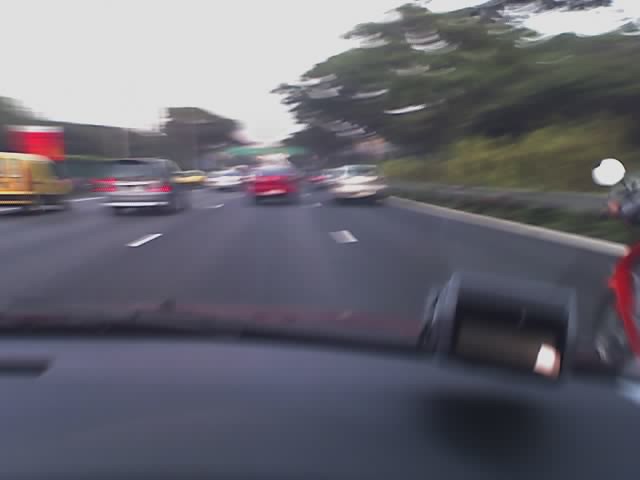The image captures a scene viewed from inside a fast-moving car, with a black dashboard and windshield wiper visible. The blurred setting depicts a large, multi-lane highway with clearly marked white dashed lines and a solid white line on the outer edge. Out of the windshield, four cars are traveling in the same direction: a white car, a red car, a gray car, and a yellow van spread across the lanes. To the right of the highway, an embankment rises with a guardrail, trees, bushes, and grass, while a concrete barrier separates opposing traffic on the left. The scene is set under a gray, overcast sky, with a hill and additional trees in the background. Ahead, a bridge and a large building are faintly visible, accentuating the outdoor setting. The overall blurry quality of the image suggests rapid movement.